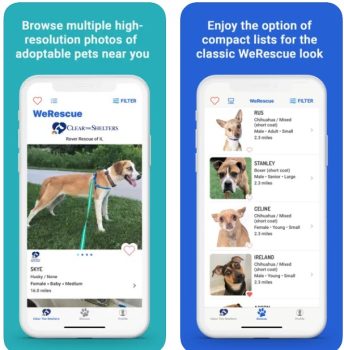The image consists of two vertical mobile screenshots, each enclosed within a blue outline. The first screenshot features a sky-blue background and promotes the browsing of multiple high-resolution photos of adoptable pets nearby. Displayed on the mobile screen is an app interface labeled "We Rescue," showcasing a profile picture of a dog standing sideways, adorned with a collar and a harness. Below the image, text likely indicating the dog's name, age, and location is partially visible but not legible.

The second screenshot has a royal blue background, advertising the option to enjoy compact lists for the classic "We Rescue" look. The mobile screen displays four thumbnail images of various dogs with brief descriptions on the right side. The first dog appears to be a large Chihuahua mix, followed by a Boxer whose partial name "Stanley" is visible. The third thumbnail shows what seems to be an older Chihuahua, and the fourth image features a dog that looks like a cross between a Chihuahua and a German Shepherd. However, the accompanying text for these thumbnails is largely indiscernible.